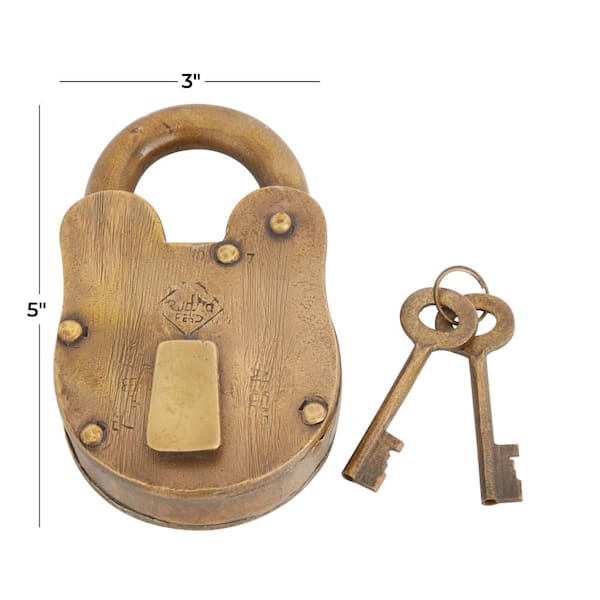The image depicts an antique Linton Lane padlock with a brass finish, prominently placed on a stark white background. The padlock is a light brown, resembling wood texture, with a distinctive arching metal shackle at the top. The front plate features five brass rivets: two in the bottom left corner, two in the upper right, and one in the bottom right corner. A lighter-colored flat rectangular area is centered on the lock, which is embellished with various markings. Notably, a black line runs vertically on the left side, marked with the height "five inches" at the top. Another black line runs horizontally across the middle, indicating the width of "three inches." There's a number 7 stamped into the lock, alongside a rectangular brass cover above the keyhole, with an inscription that's partially readable as "rudra something fend." On the right side of the image, a pair of brass skeleton keys, connected by a small ring, accompany the padlock. The overall color palette includes shades of tannish beige, black, and white, accentuating the antique and detailed nature of the items.